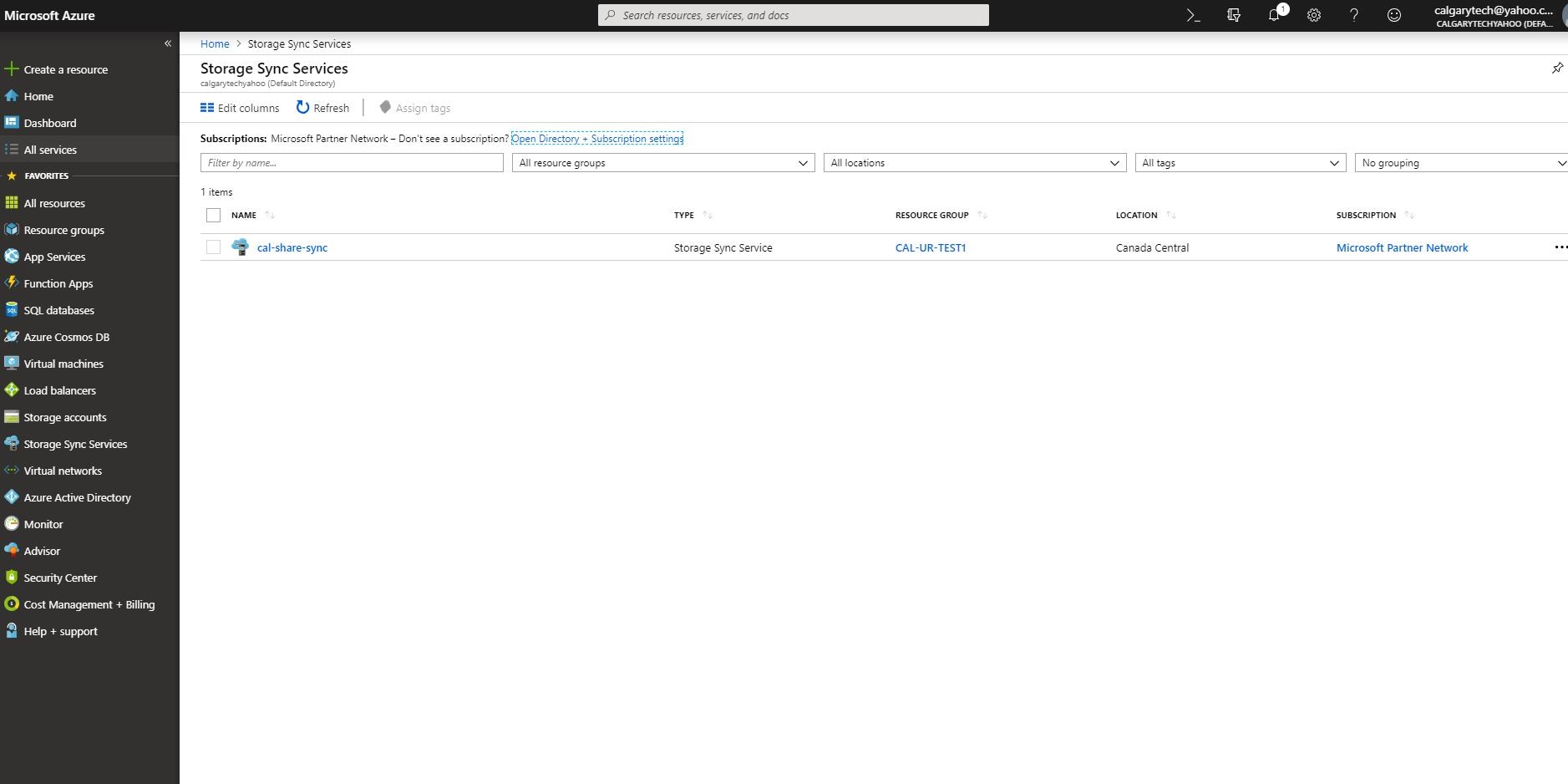The webpage displayed is the Microsoft Azure portal, easily identifiable by the "Microsoft Azure" text in white lettering located in the top-left corner. Dominating the left side, a vertical navigation bar with a black background features a series of icons and labeled menus. These include categories such as "Create a Resource," "Home," "Dashboard," and "All Services," followed by a section labeled "Favorites" with additional items listed underneath.

The main content of the page is focused on "Storage Sync Services." Positioned below this header is a search area designed to filter subscriptions by name. At the upper section of the main content area, a row of horizontal drop-down menus allows for filtering by various criteria including "All Resource Groups," "All Locations," "All Tags," and "No Grouping." These menus facilitate navigation and the organization of resources.

Directly beneath these filters, a single entry appears, presumably a subscribed service, displayed as a hyperlink in blue text reading "CAL-SHARE-SYNC."

In the top-right corner of the webpage, user account information is partially visible, indicating that someone is logged in with an email address starting with "calgarytech@yahoo.com," though the full address is truncated.